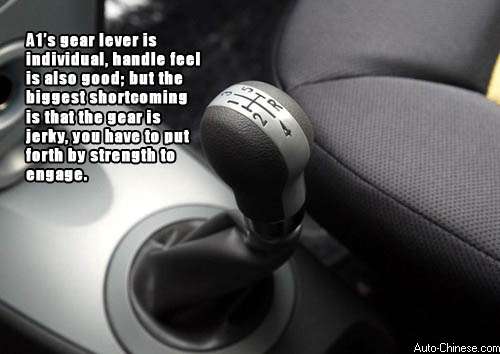The image is a detailed, color photograph in landscape orientation, showcasing the interior of a car, specifically focusing on the gear shift. The central subject is the car's manual gear lever, prominently positioned in the middle of the frame. The gear shifter is black with a silver stripe running across its top, displaying the gear pattern in black. Encasing the gear lever is a black vinyl or leather boot that fits snugly into a circular opening in the sleek, silver chrome console.

To the left of the gear shift, white text reads: "A1's gear lever is individual. Handle feel is also good, but the biggest shortcoming is that the gear is jerky. You have to put forth by strength to engage." This text succinctly describes the usability of the gear lever, focusing on both its positive and negative attributes.

Towards the top right of the image, part of the passenger seat is visible. It features a dark gray upholstery with a hint of a gold center panel, adding a touch of contrast to the interior's predominantly monochromatic palette. The colors in the image are primarily black, dark gray, light gray, silver, and white. The bottom right corner of the image contains the website watermark, "autochinese.com," indicating this is likely an informational photograph meant for a blog or car review website. The entire composition blends realism with typographical elements, providing both a visual and descriptive understanding of the car's manual gear shift.